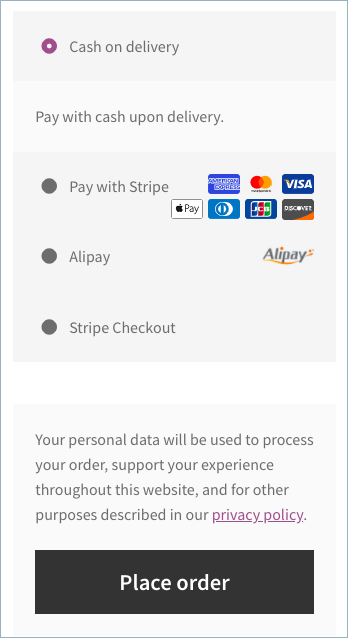The image appears to be a vertical screenshot from a mobile phone displaying a payment page for an online transaction. At the top, a gray horizontal bar spans the width of the screen, containing the text "Cash on Delivery." This option seems to be selected, as indicated by a purple button to its left. Directly below, in a white section, the text "Pay with cash upon delivery" is displayed.

Further down, the options "Pay with Stripe," featuring multiple credit card icons to its right, "Alipay" with its corresponding symbol, and "Stripe Checkout" are listed in a gray area, each marked with an unselected gray dot.

The selected "Cash on Delivery" option is highlighted in purple, while the other payment methods remain unselected in gray.

Beneath the payment options, black text on a white background informs users that their personal data will be used to process the order, support their experience on the website, and fulfill purposes outlined in the privacy policy.

Finally, at the bottom of the screen, a large black rectangle labeled "Place Order" in white text serves as the button to finalize the purchase.